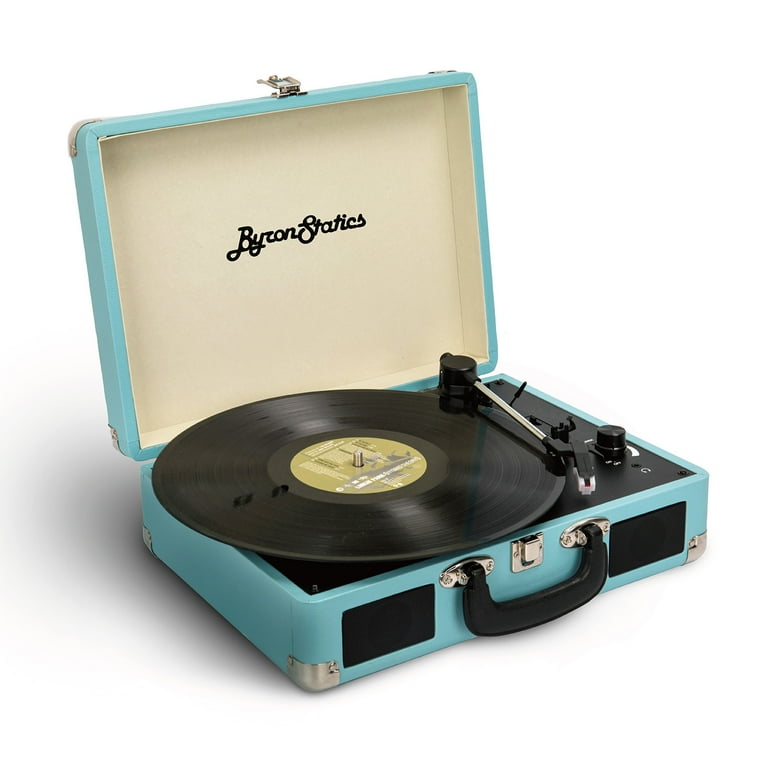The image showcases a portable, vintage-style record player designed like a suitcase, allowing it to be carried easily from place to place. The exterior of the suitcase is a charming light blue, also described as turquoise, and features a black handle with a lock mechanism in the front. The sides of the handle are adorned with decorative black squares, likely housing the built-in speakers. 

When opened, the top lid of the suitcase reveals white lining with the brand name, "Byron Statics," elegantly written in cursive black lettering. The main compartment houses the record player, which includes a black turntable with a gold center, currently holding a record. The arm of the record player, equipped with a needle, is positioned at the start of the record, indicating it’s ready to play.

To the right of the turntable, built into the suitcase, is a black volume control knob and a plug for headphones, indicating the record player is equipped for private listening. The entire unit appears to be battery-operated, as no cords are visible, making it truly portable. Silver embellishments decorate each corner of the suitcase, adding a touch of vintage elegance to the design.